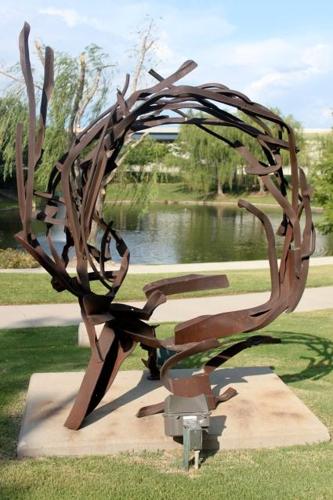The photo features a striking piece of modern art situated in a picturesque park. The artwork, crafted from forged iron and steel, forms a large, complex, globular structure resembling a planet or abstract globe with various metallic extensions protruding from it. This sculpture rests on a concrete slab and appears to include lighting at its base for nighttime illumination. In the foreground, well-manicured grass leads to a walking or biking trail made of concrete. Further in the background, a serene pond surrounded by lush trees and bushes completes the scene, all beneath a sky dotted with white clouds. The entire setup exudes a tranquil, pastoral vibe, underlining the harmony between modern art and natural beauty.